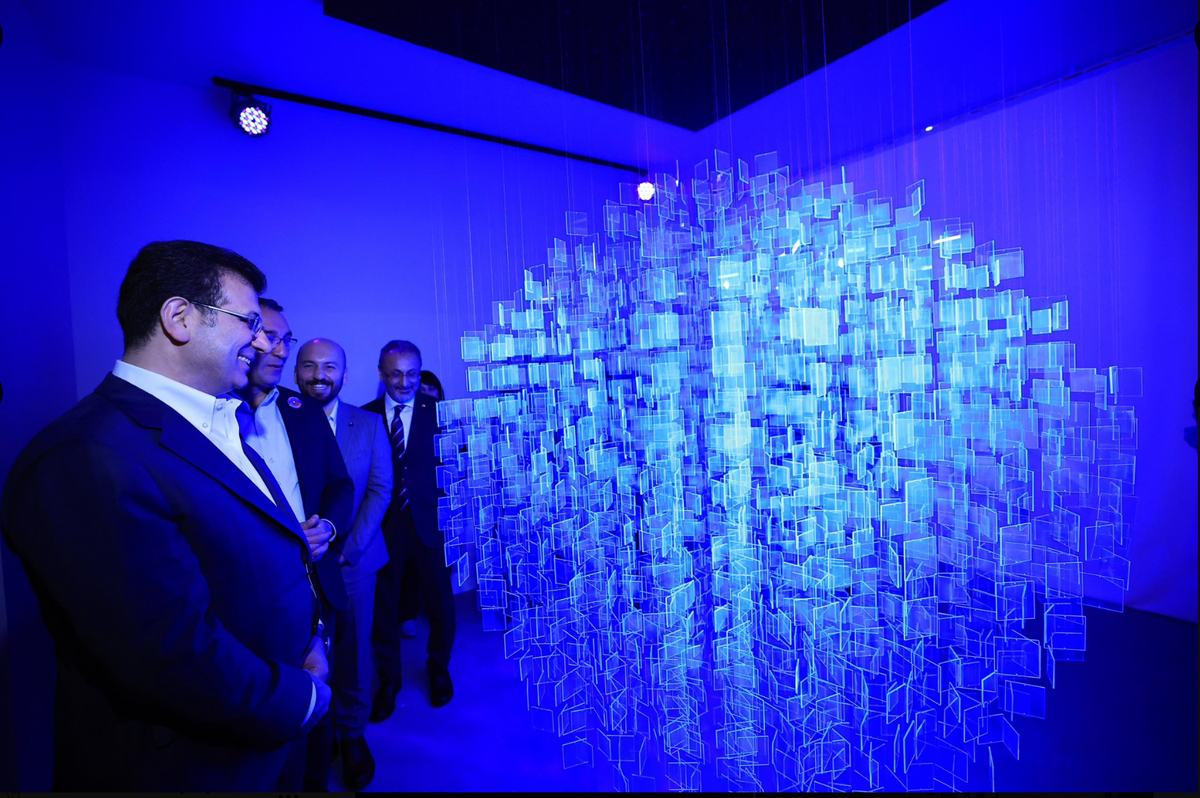In this indoor photograph, a group of individuals is gathered in a room with high ceilings, thoroughly illuminated by rich blue and slightly purple hues. The focal point of their attention is a striking art installation in the center, resembling a chandelier but distinctly modern in design. This installation, made up of countless rectangular crystalline or glass panels, forms a large suspended sphere. The sphere is composed of disjointed panels with a turquoise and light blue coloration, interspersed with white highlights, giving it a glittery appearance.

The sphere is held aloft by a black bar affixed to a blue wall behind it, although the exact mechanism of its suspension remains ambiguous. Surrounding the installation, the men, dressed in dark suits and white shirts with varying accessories, are arranged in a queue on the left side of the frame. The man in the foreground, possibly middle-aged with dark hair and wire-rimmed glasses, wears a dark blue suit jacket over a white button-down shirt, appearing engaged and smiling at the installation. Behind him is an assortment of men of different ethnicities, including an African man with a full beard and a South Asian man, all intently observing the art piece and seemingly impressed by its intricate construction and luminous beauty. The room's ceiling adds to the atmosphere with its black surface contrasting the vivid blue lighting.